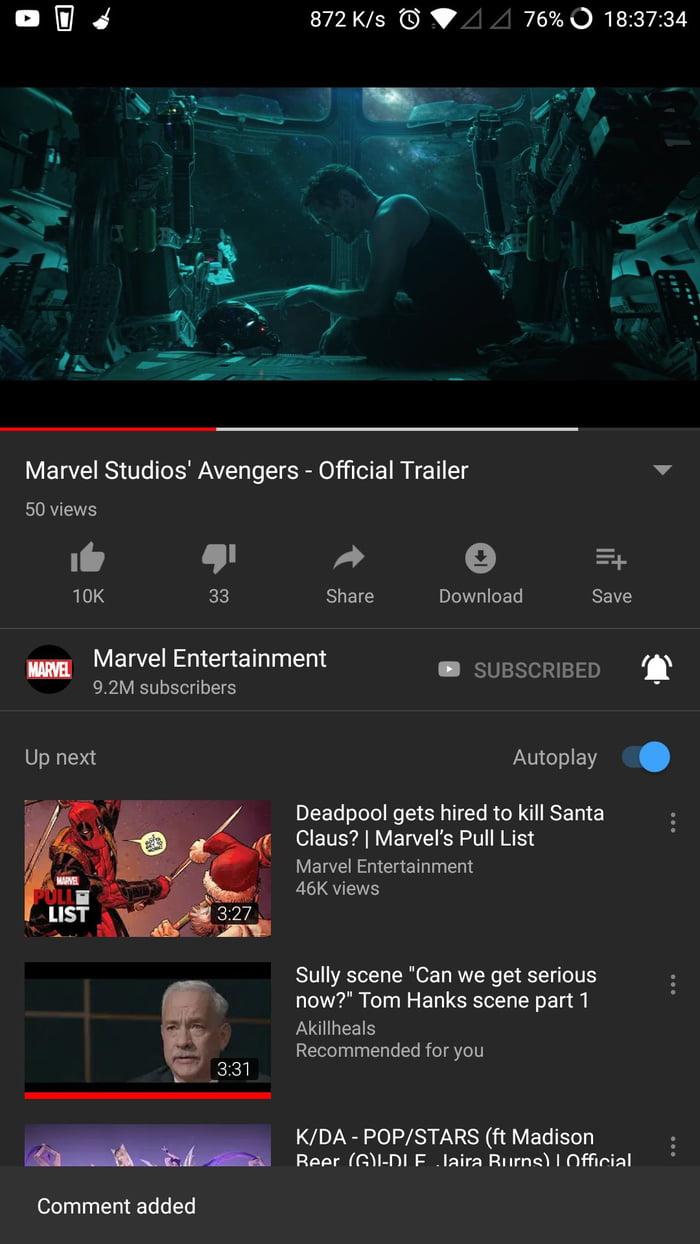The screenshot captures a YouTube video interface on a mobile device in dark mode. The background is a deep gray, almost black, with white text and icons. The top status bar displays an 872K/s data rate, a clock, fully connected Wi-Fi signal, and a battery percentage of 76%. The time is noted as 18:37:34.

The main content area showcases a scene from a Marvel Studios production where a character is gazing downward, seemingly at an Iron Man mask. Below this scene is the red progress bar which indicates that the video is partially played, with a loaded portion highlighted in white that does not yet span the full width of the screen.

The video identified in the screenshot is titled "Marvel Studios' Avengers Official Trailer," with 50 views, 10K likes, and 33 dislikes. Buttons for sharing, downloading, and saving the video are present, and the channel "Marvel Entertainment" is shown to have 9.2 million subscribers with the user subscribed.

Beneath the main video player, the "Up next" section lists a video titled "Deadpool Gets Hired to Kill Santa Claus | Marvel's Pull List" from the same channel. This next video has 46K views and is 3 minutes and 27 seconds long. Text indicating additional recommended content follows, including a video titled "Tom Hanks Scene Part 1" by Akili Hills, lasting 3 minutes and 31 seconds.